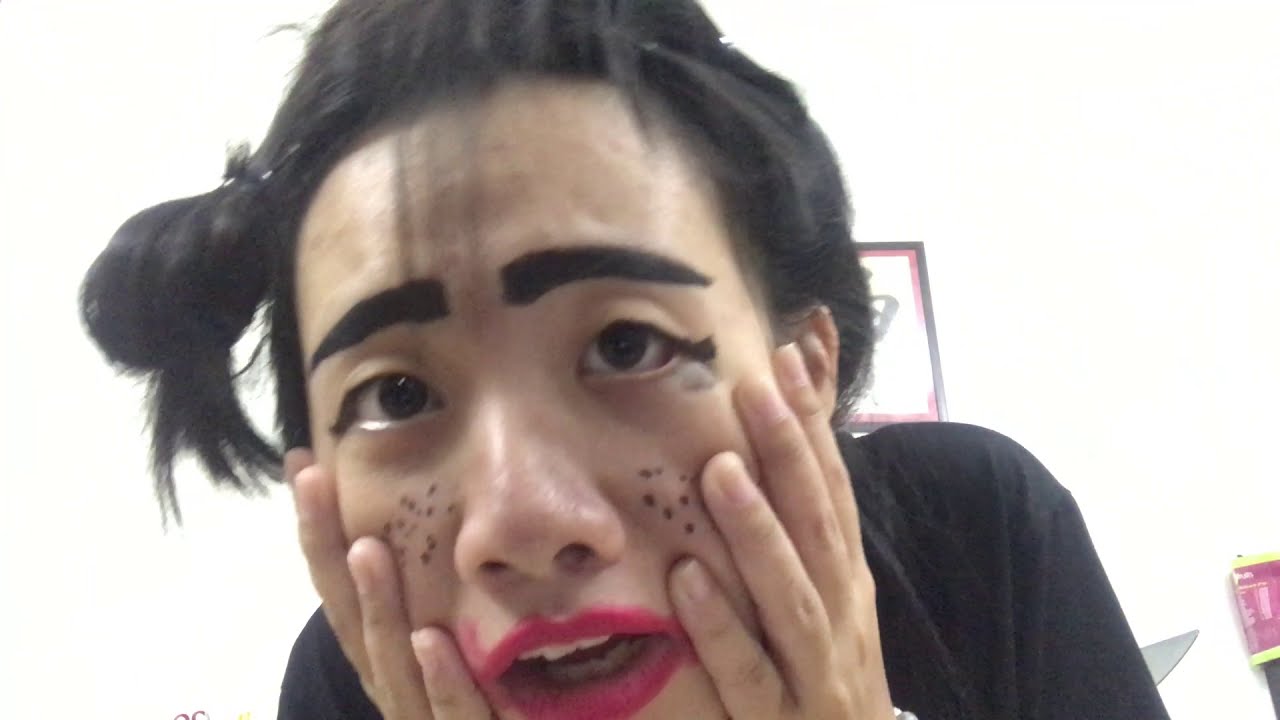The photograph features a close-up of an Asian woman in her mid-30s, indoors against a stark white wall. Her dark hair is styled into a side bun secured with a clip, with a few strands falling across her forehead. Her face, framed by her hands pressing against her cheeks, displays dramatic makeup: smeared bright red lipstick extending beyond her natural lip line, exaggerated and filled-in black marker eyebrows resembling caterpillars, and artificial freckles dotted on her cheeks. Her eyes, accentuated by heavy mascara and extended black eyelashes, stare intensely at the camera. Her mouth is slightly open. She wears a dark top. In the background, a barely visible framed picture peeks out from behind her, contributing to the visual details of the indoor setting.